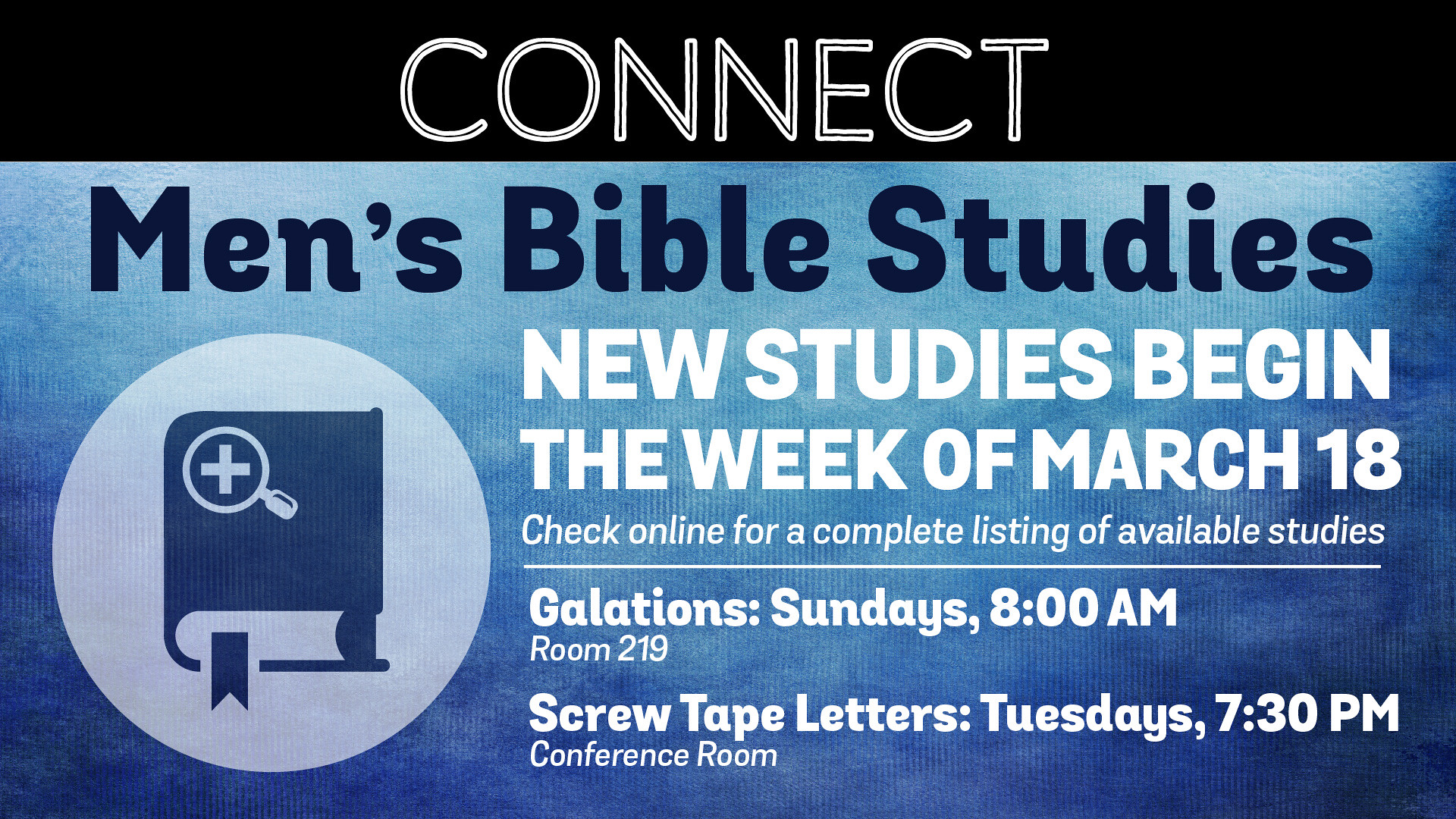The image is a poster advertising an event related to Men's Bible Studies. The top portion features a horizontal black strip with the word "Connect" written in white. Below, the text announces that new studies will begin the week of March 18 and advises checking online for a complete listing of available studies. It highlights two specific studies: Galatians on Sundays at 8:00 a.m. in room 219, and The Screwtape Letters on Tuesdays at 7:30 p.m. in the conference room. On the left side, there is a circular logo featuring a book with a magnifying glass, and a cross, with a bookmark sticking out. The background of the poster transitions from dark blue at the top to light blue towards the bottom, with most of the text written in white on top of the blue background.